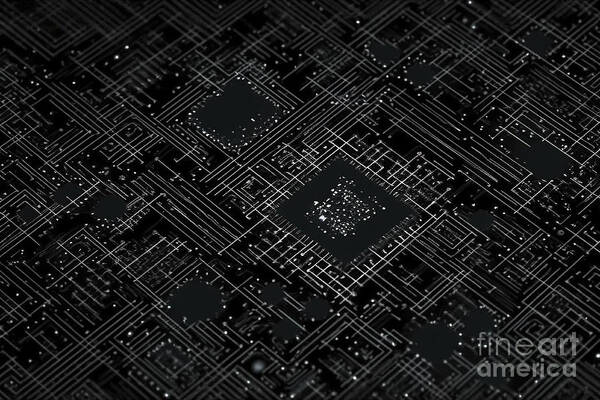This is a striking black and white abstract artwork that evokes the intricate design of a computer's circuit board or motherboard, suggesting multiple microprocessors and the intricate connections between them. The composition uses varying shades of gray, from light to dark, with the circuit-like lines rendered in white, creating a stark contrast that enhances the intricacy of the schematic-like patterns. Central to the image is a figure reminiscent of a CPU, surrounded by a complex web of fine lines that resemble the array of connections within a computer system. The bottom right corner of the image bears the words "Fine Art America," indicating its artistic intent. This versatile piece, which could also be interpreted as a night sky filled with stars and delicate webbing, ultimately stands out as a unique and captivating example of abstract art.